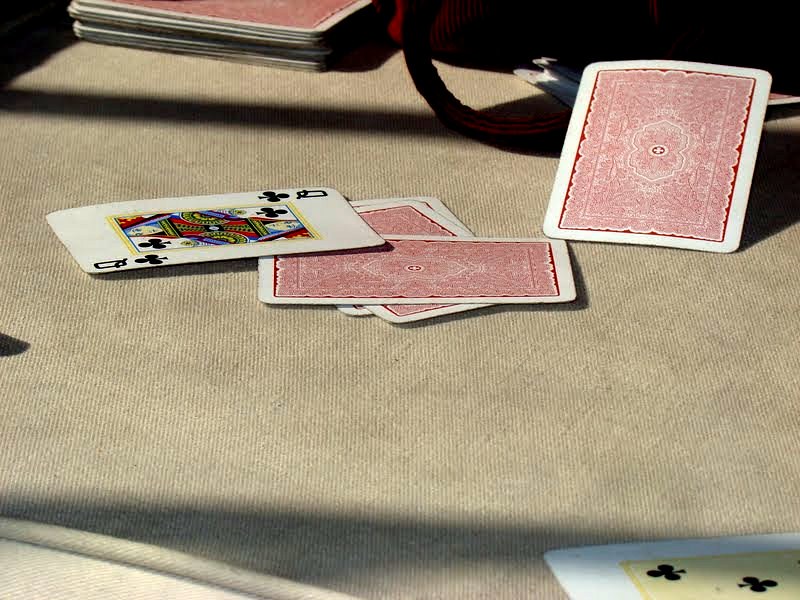In this full-color landscape-oriented photograph, the scene features a khaki-colored tablecloth with a burlap-like texture, illuminated by sunlight that casts shadows both in the forefront and background. The primary focus of the image is a collection of playing cards arranged at the center. At the heart of this arrangement are four cards stacked together: two cards face down in a vertical alignment, one card placed horizontally across them, and on top of this lies the face-up Queen of Clubs. The Queen of Clubs card is white with black markings for the suit, while the queen's image itself is rendered in red, blue, and yellow.

To the right of this central stack, a single face-down card is visible. Partially revealed in the lower right corner of the image is the top corner of a club-suited card, although its rank is indiscernible from the visible portion. In the top left corner of the photograph sits the remainder of the deck, face down, showcasing a white border and a red intricate design on the back of the cards. Additionally, situated in the center top of the image is a mysterious half-circle shape whose purpose is unclear.